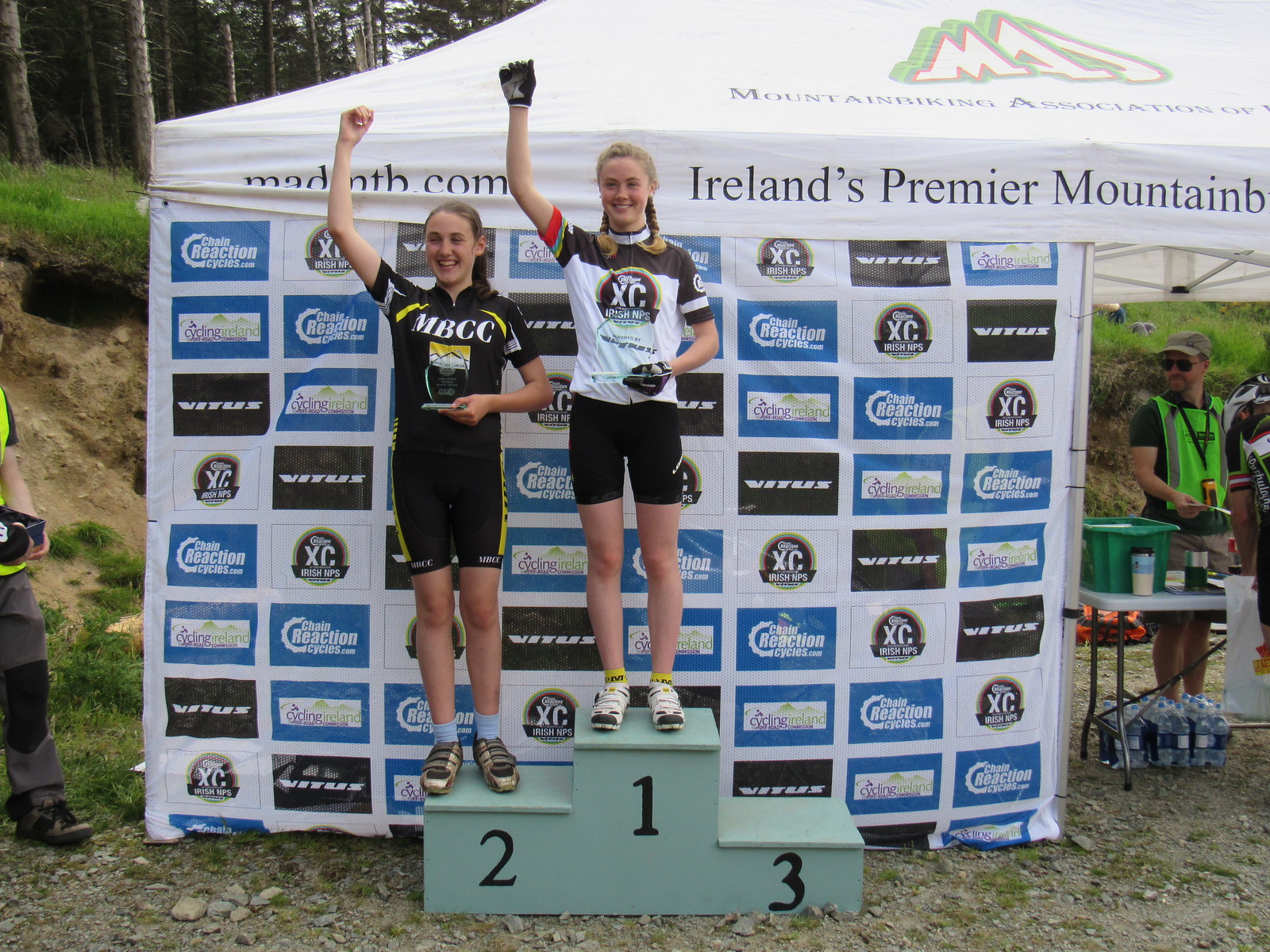In this large square image, two teenage girls, presumably mountain bike racers, stand on a podium under a tent that reads "Mountain Biking Association, Ireland's premier mountain biking" (partially obscured). The podium has three steps marked 1, 2, and 3, with the numbers indicating ranking positions. The girl occupying the number one spot wears a white and black jersey with the letters "XC" on it, black shorts, and black gloves. She raises her right hand high above her head. To her left, standing on the number two step, is another girl in a black, white, and yellow jersey with "MBCC" printed across her chest and black shorts. She also has her right hand raised, while her left hand is bent at the elbow holding an indistinguishable object. Both girls have blondish-brown hair pulled back. The backdrop features a variety of sponsor advertisements, including Chain Reaction Cycles and XC Irish NPS, and showcases the outdoor, rocky and weedy terrain typical of a cross-country setting. Inside the tent, a man in a bright green vest appears to be providing refreshments.